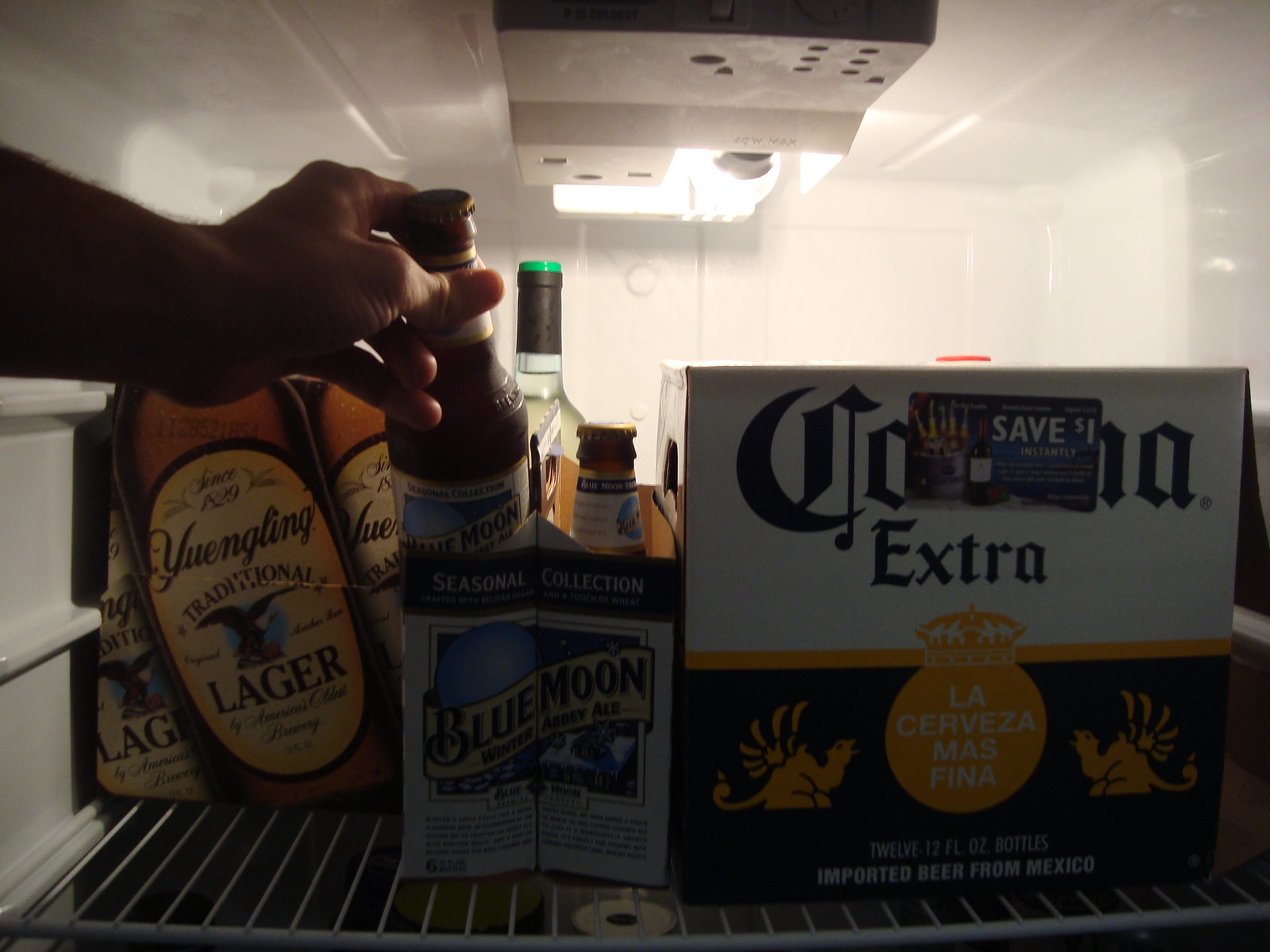Inside the well-lit top shelf of a refrigerator, a person is seen reaching for a Blue Moon Winter Abbey Ale bottle from a six-pack situated in the center. The Blue Moon bottles are brown with tan and blue labels. On the left side of the shelf, there is a box of Yuengling Traditional Lager, clearly labeled with "Yuengling" and "Since 1829". On the right side, a 12-pack box of Corona Extra is prominently displayed, featuring a white, gold, and yellow design with a crown, two dragons, and "La Cerveza Mas Fina" written on it. The Corona box also has a sticker indicating a one-dollar savings offer. Behind the Blue Moon box, a partially visible glass bottle with clear liquid and a black top suggests the presence of another type of liquor, possibly vodka. The refrigerator’s wire rack and its light fixture add to the organization and visibility of the scene.